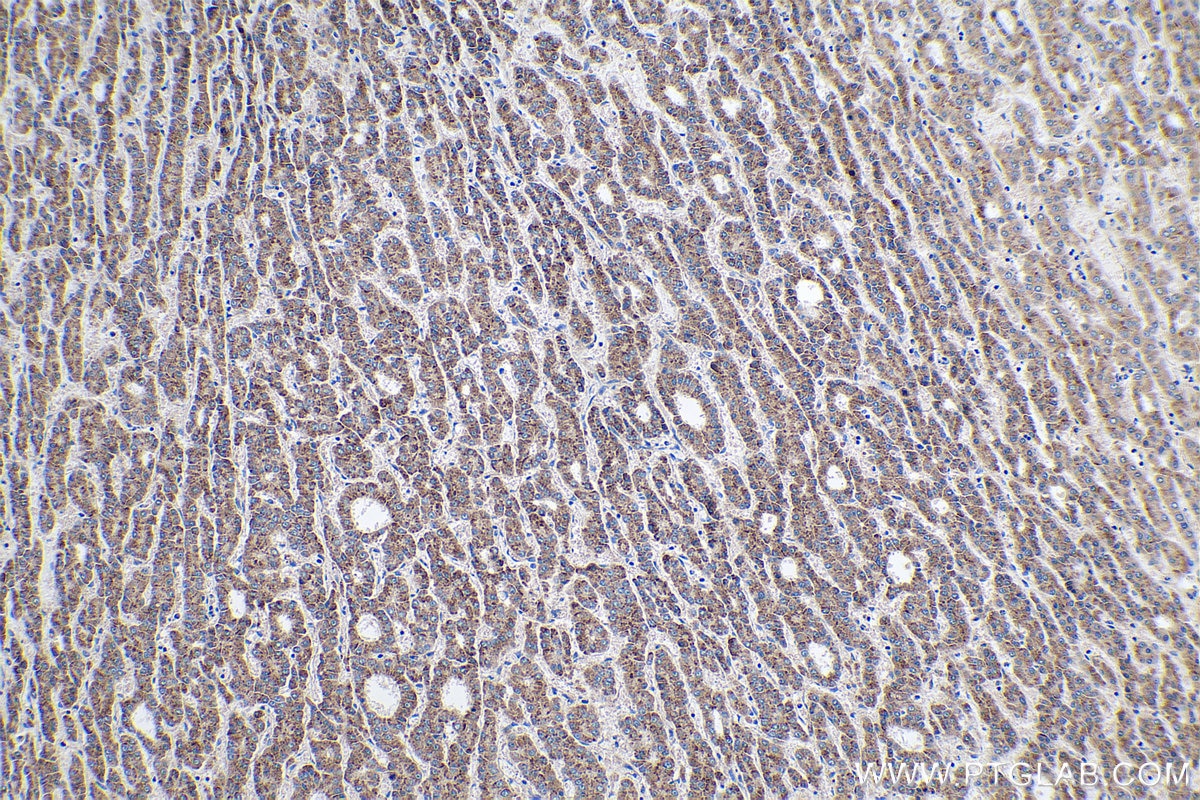This detailed landscape-oriented photograph, featuring a watermark that reads "www.ptglab.com" in the bottom right-hand corner, captures a close-up view of microscopic objects. The image palette primarily consists of light gray, brown, and white hues. Scattered across the photograph are circular objects interspersed with darker, cylindrical shapes. These cylindrical structures appear to run diagonally from the top left to the bottom right, creating an intricate pattern that draws the viewer's eye along this dynamic trajectory.